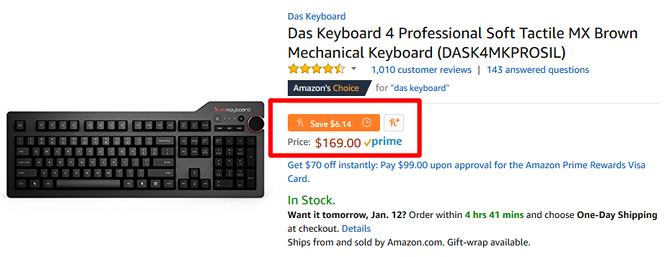This is an online advertisement for a DOS Keyboard, featured on a webpage that does not specify the hosting website but displays the Amazon's Choice logo. The product advertised is the DOS Keyboard for Professional Soft Tactile MX Brown Mechanical Keyboard (model: DASK for M-K-P-R-O-I-S-I-L). It boasts a customer rating of 4.5 stars based on a thousand reviews, indicating high user satisfaction.

The advertisement mentions the pricing and discounts available. The keyboard is priced at $169 on Amazon Prime. Notably, shoppers can save $6.14 by using the Honey browser extension. Additionally, there is an offer to get $70 off instantly, bringing the price down to $99 upon approval for the Amazon Prime Rewards Visa Card.

The stock status confirms that the keyboard is available for immediate purchase, with options for expedited shipping. Customers who place their order within four hours and 41 minutes can opt for one-day shipping and receive the item by January 12th. The product is shipped from and sold by Amazon.com, with gift wrapping options available.

The accompanying image depicts the keyboard, which has a standard, straightforward design with a few additional buttons located in the top right-hand corner. The ad reflects mixed sentiments, with the narrator expressing reluctance to pay $170 for the keyboard despite the detailed listing and various promotions.